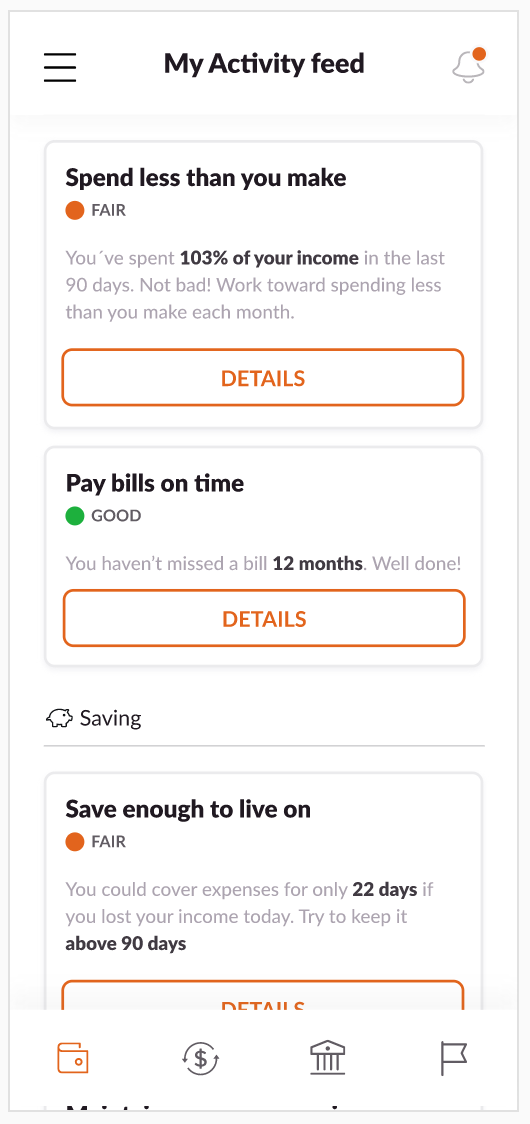This is an image depicting a detailed financial tracking app interface, presented in a long rectangular format typical of mobile applications. 

At the very top of the interface, there's a heading titled "My Activity Feed." Directly beneath it, there's a section labeled "Spend Less Than You Make." This section outlines the percentage of income spent over the last 90 days, stating, "You spent 103% of your income in the last 90 days." The "103% of your income" is bolded for emphasis, likely to draw immediate attention. Below this statement, there is an orange rectangular link labeled "Details" which users can click for more information on managing their spending.

The middle section is devoted to the user's progress on "Pay Bills On Time." The heading is in black text, and the user's status is marked as "Good" with a green dot indicator, followed by the congratulatory summary, "You haven't missed a bill in 12 months. Well done." The "12 months" is prominently bolded. This section also includes an orange rectangular button for further interaction.

The final section covers savings, under the heading "Save Enough to Live On" in black text. The app informs the user that their status is "Fair," stating, "You could cover expenses for only 22 days if you lost your income today. Try to keep it above 90 days." Both "22 days" and "90 days" are bolded to stress these critical numbers. This section serves as a cautionary alert highlighting the user's current financial vulnerability.

At the bottom of the app interface are four symbols: an orange wallet, a black dollar sign surrounded by two arrows, a black bank icon, and a black sign/banner. These icons likely represent different interactive features or sections within the app.

Overall, this financial app menu provides a comprehensive overview of the user’s spending, bill payment, and savings progress, along with actionable insights and interactive elements to help improve financial health.